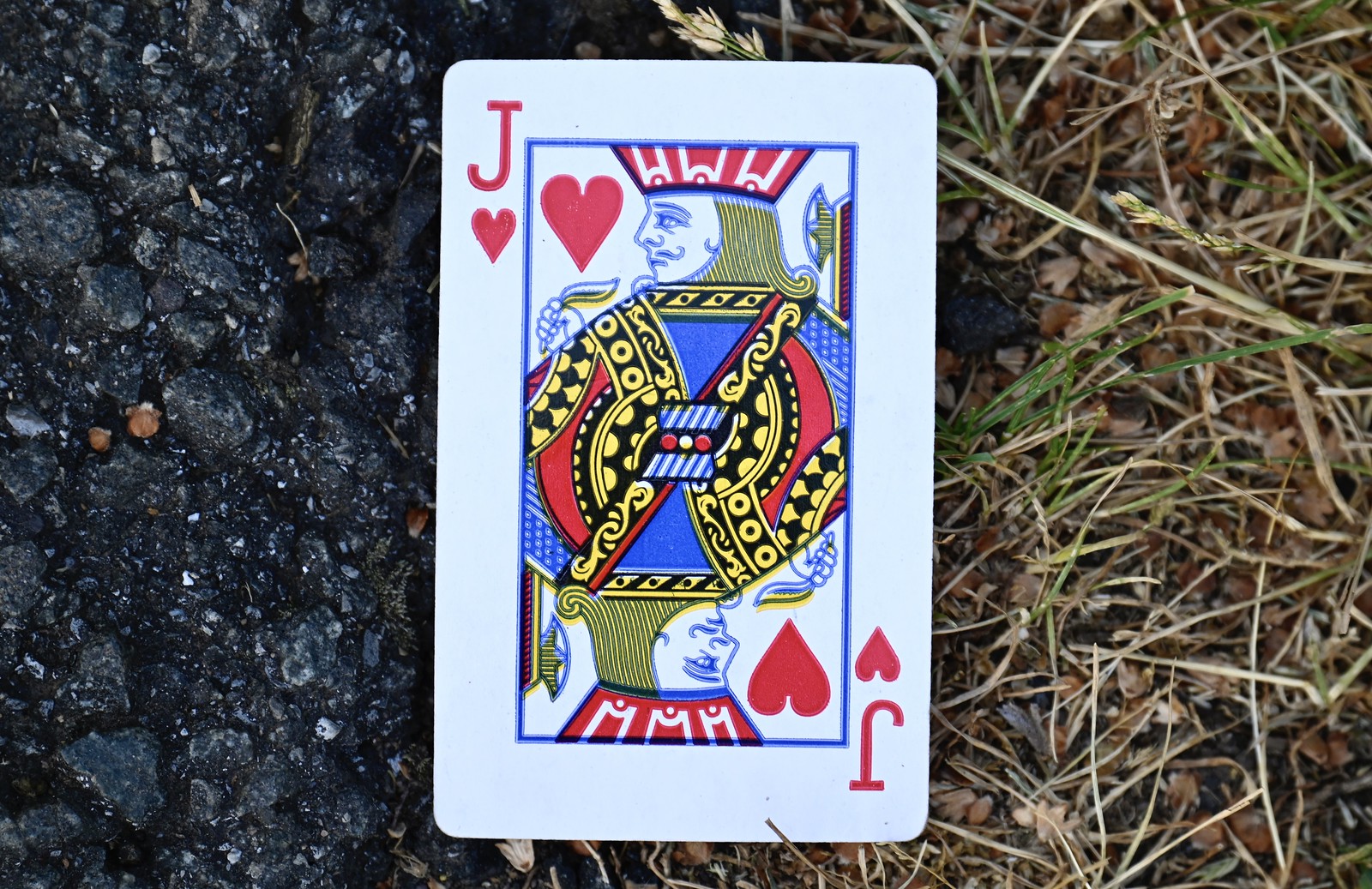This photograph features a single white playing card, specifically the Jack of Hearts, lying on the ground. The card is positioned such that one half rests on a stretch of asphalt, while the other half lays over a patch of grass that is partly green and partly brown. The Jack of Hearts card showcases the traditional mirrored image design: a red "J" and red heart symbol are present at both the top and bottom of the card, which are connected by a blue rectangular border. Inside this border, the Jack of Hearts depicts an ornate, vibrant illustration of a man wearing a red hat, adorned with long, blonde, curly hair that curls at the ends. The man is shown holding an axe and is dressed in elaborate robes, capturing the classic and distinguished appearance typical of a face card.